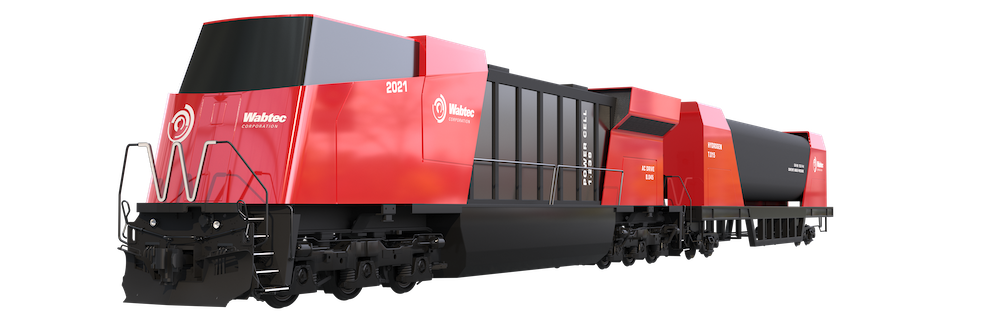A highly detailed and futuristic photograph, possibly a 3D render, depicting a modernistic Wabtec locomotive. The train moves from the upper right to lower left on an all-white background, emphasizing the sleek design of the electric or hydrogen-powered engine. The front cab, positioned to the lower left, features a glossy black, wraparound window, providing an ultra-modern aesthetic.

Prominently, the front end of the train is red with white letters spelling out "WABTEC," and the year "2021" displayed on the side. The cab is equipped with an aluminum guardrail shaped like a W, which is bordered by steps leading up to the entry. Below, the black undercarriage shows hints of the train's wheels.

The middle section of the train contains a distinct black segment inscribed with "POWER CELL 1," indicating a possible energy source. Following this is another red section repeating the "WABTEC" branding. The rear includes another black segment, ending with a slimmer, red part. This ultra-modern train is likely a conceptual image for a hydrogen or electric-powered locomotive, reflecting cutting-edge advancements in sustainable rail transport.